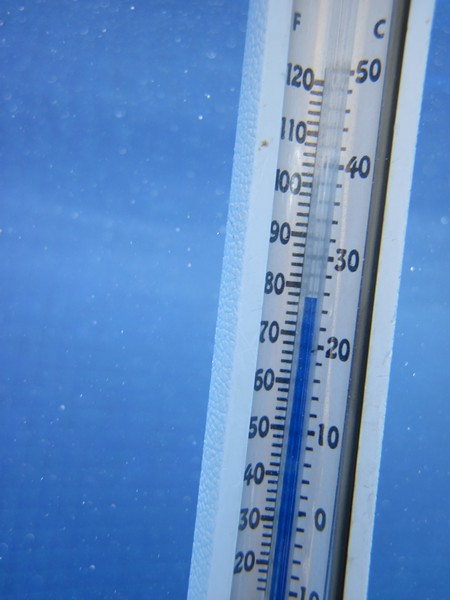The image is rectangular with a vibrant blue background, resembling droplets of moisture scattered across it. Positioned slightly off-center towards the right and running diagonally from top to bottom, there are two thermometers incorporated into a single unit. One thermometer is marked with an "F" for Fahrenheit, while the other is labeled with a "C" for Celsius. Both thermometers share a central blue fluid column that provides the temperature reading. The current temperature displayed is 78 degrees Fahrenheit and 35 degrees Celsius. The exact location or context of the thermometer is not apparent.